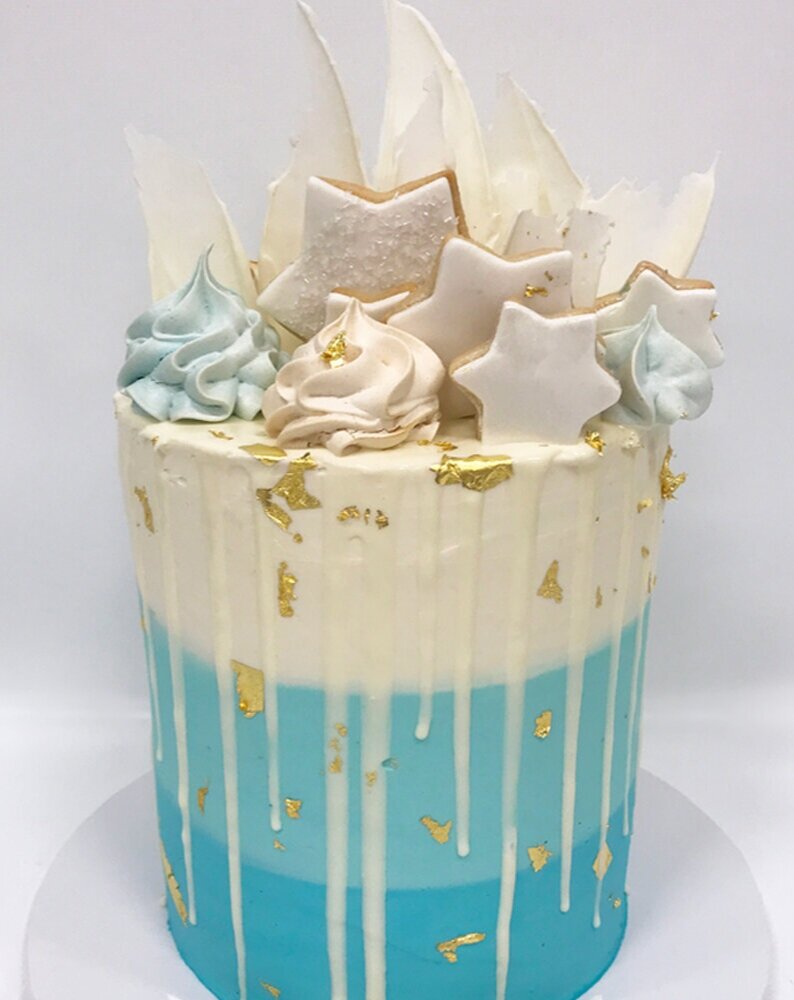The image features a photorealistic, three-layered dessert that alternates between teal, sky blue, and off-white tiers, reminiscent of a wedding or bridal shower cake. Set against an off-white to grayish background, the dessert sits atop an off-white cylindrical platform that’s slightly raised from the ground. Drips run down its sides, heightening the photorealistic touch. The top layer of the dessert is adorned with star-shaped cookies and an array of rosettes and flowers made of frosting or whipped cream, arranged as if squeezed out of a confectioner's bag. Some elements resemble large toasted coconut flakes, adding texture to the elaborate design. The star-shaped cookies are partly embedded in the dessert, creating a visually striking and dramatic effect. Overall, the detailed and attractive presentation suggests the dessert or its artistic imitation could elegantly grace a special occasion.